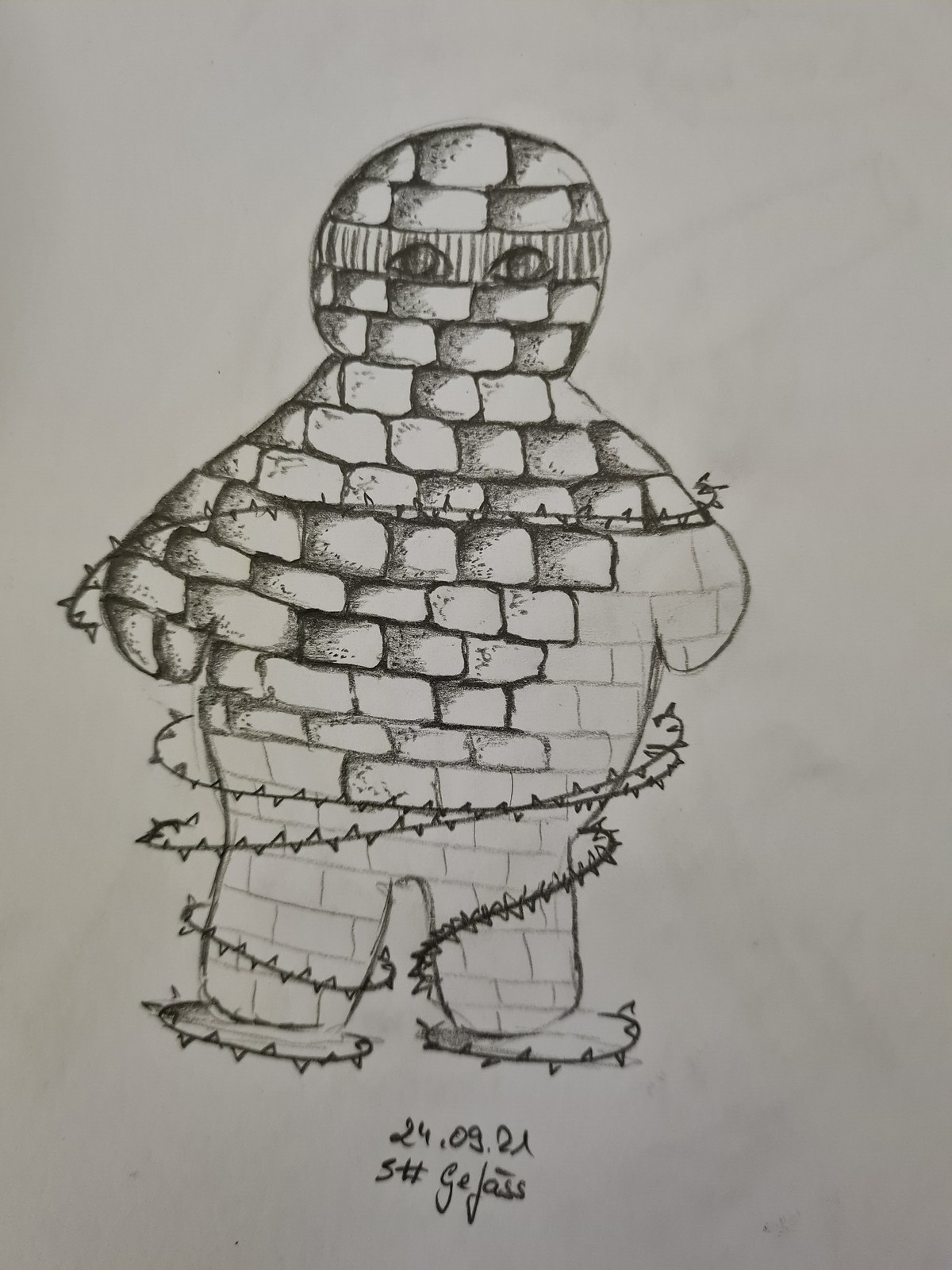This detailed illustration on white construction paper features a humanoid character rendered entirely in black and white. The character's head and upper body resemble the texture and arrangement of igloo bricks or castle stones, giving it a robust and stony appearance. The character is bald and has two prominent eyes located near the top of its head. Barbed wire encircles the figure, especially around the legs, adding a sense of confinement or danger. The characters’ feet are adorned with shoes that have spikes protruding from them, enhancing the menacing aura.

At the bottom of the illustration, there is black text that reads "24.09.21," possibly indicating a date. Below this date, a name is inscribed, which appears to be "STTGOJASS" or a similar variation. The overall style of the drawing evokes an image of a Pillsbury Doughboy if it were constructed from castle-like stones and encased in barbed wire, blending an unusual mix of innocence and stark ruggedness.